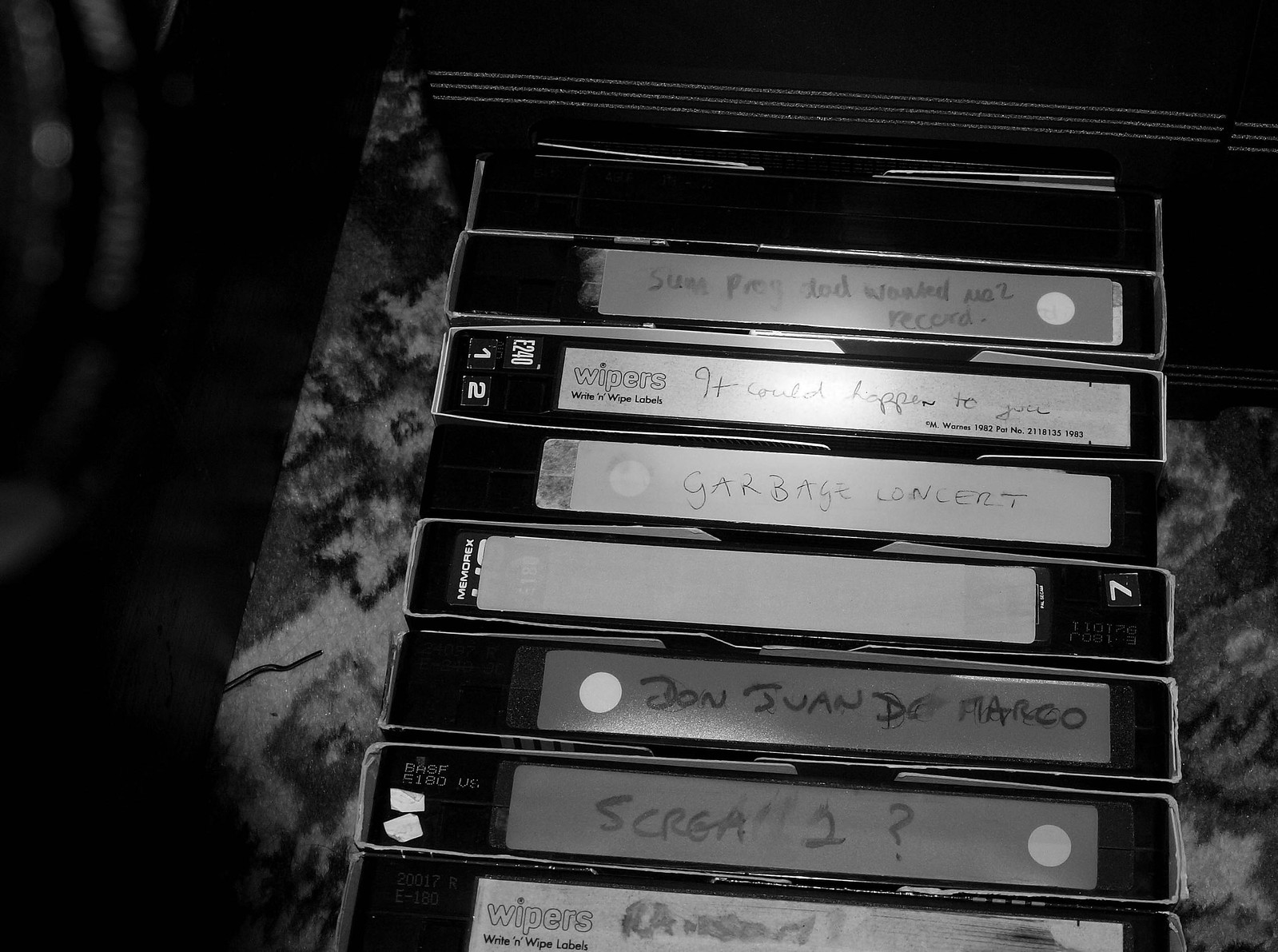This black and white photo captures an array of approximately ten old VHS tapes, meticulously laid out in parallel positions, allowing clear visibility of their white labels. The tapes rest on what could be a blanket, carpet, or possibly a tie-dye-like floral cushion, adding a nostalgic touch to the scene. Among the handwritten labels, some are distinctly legible, contributing to the tableau of personal history encapsulated in these recordings. The labels feature intriguing titles such as "Some Pray / Dad Wanted," "It Could Happen to You," "Garbage Concert," "Don Juan DeMarco," and "Scream 2?"—the latter showing signs of smearing. One tape notably lacks a label, while another's inscription appears partially erased, invoking a sense of bygone eras and forgotten memories. This evocative arrangement vividly brings back the era of VHS tapes and home recordings.